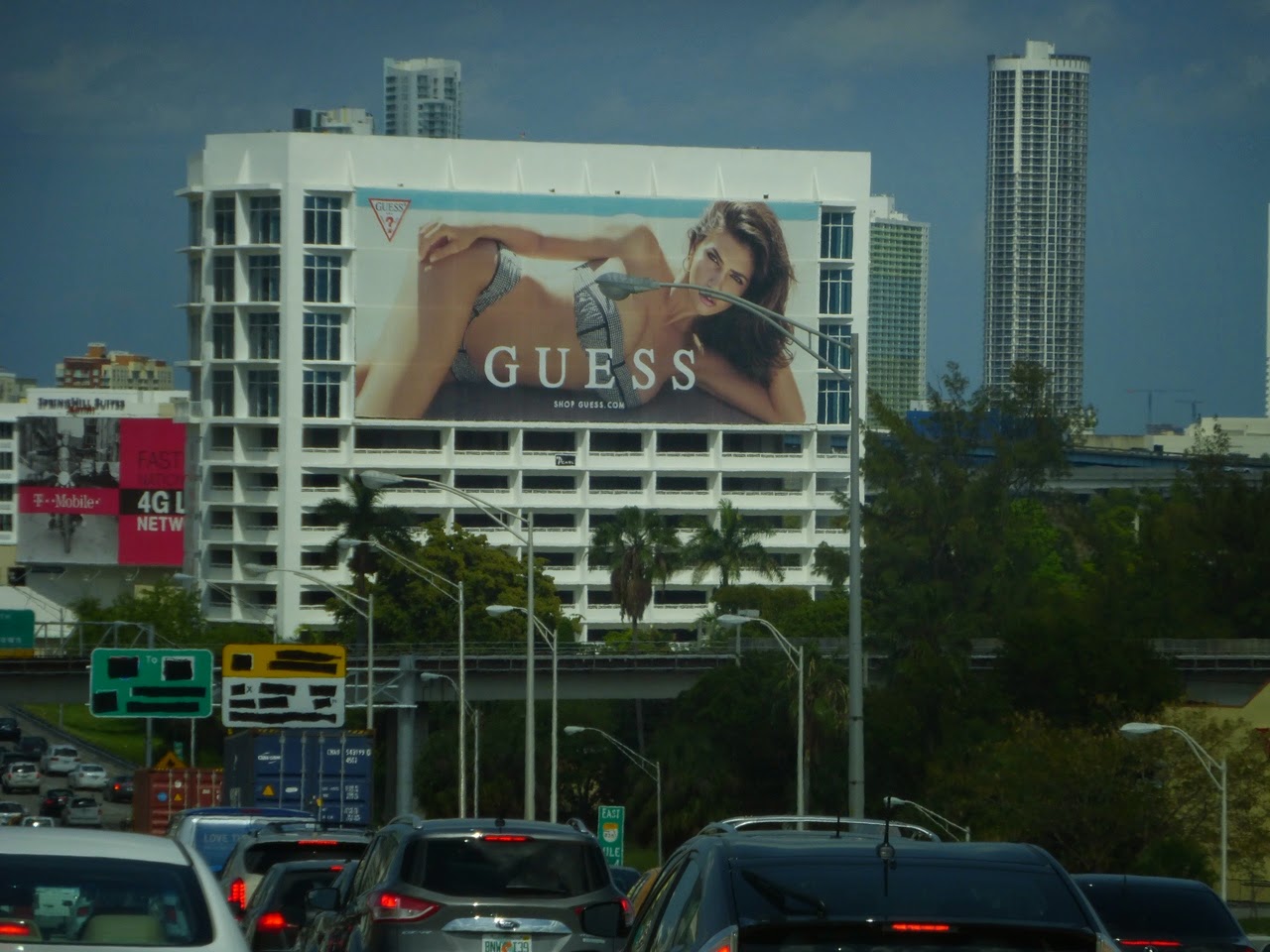In this daytime photograph, the scene is set against a bright blue sky, despite the image's graininess and lower resolution. Central to the composition is a towering white high-rise building with a somewhat oval design on its sides. Spanning four stories of the building, a colossal advertisement features a female model in a bikini with the text "Guess" and the website "shop.guess.com." The ad is prominent, with the iconic Guess logo in an inverted triangle in the upper left corner of the billboard.

Beneath this structure runs an overpass, bustling with heavy traffic, evident from the numerous cars with illuminated brake lights traveling away from the observer. Adding to the urban atmosphere, the top right corner of the photo reveals another extremely tall high-rise building. The presence of several palm trees within the scene indicates that this location is in a warm climate zone. The image, although not in the highest resolution, captures the lively essence of city life under a clear daytime sky.